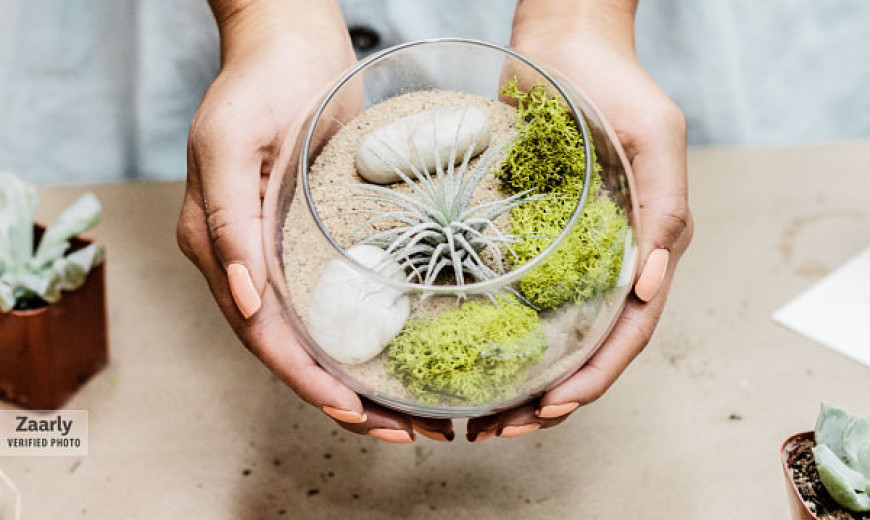This image depicts a close-up of a woman with medium to light skin holding a glass jar terrarium with both hands, showcasing her long, peach-painted nails. The terrarium contains a layer of brown, beige, grainy sand, with two beige stones, a cactus-style plant at the center, and three small green bushes along one edge. Additionally, there is some green, lime-colored moss inside the jar. The woman is dressed in a pale blue linen dress adorned with darker blue to black buttons and stands over a tan-colored table. To her left side, a small burgundy planter holds a petite plant. Light from the right side of the image reflects off her hands and the terrarium, enhancing the details of the scene.